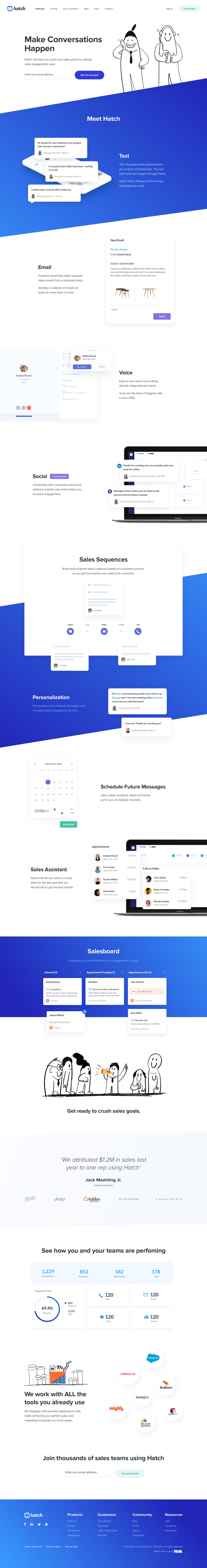The image features a series of vertically arranged screenshots set against a primarily white background, making the sequence decidedly taller than it is wide. Positioned in the upper left corner, there is a square-shaped icon with a blue background and a chunky capital letter "H" at its center. Adjacent to this icon is the brand name "Hatch." Next to the brand name are several clickable links or menu items organized into categories, including Features, Pricing, Our Customers, Blog, Help, and Contact.

On the right side of the image, a series of drawn, cartoon-like humanoid characters can be seen. These characters have a whimsical and blocky design, featuring simplistic faces with dot eyes and upturned line mouths. Some characters display distinct features, such as ponytails and headphones, adding to their individuality. Further down the image, more of these cartoon characters appear, maintaining the same stylistic attributes.

Throughout the image, multiple blue dividers are present, transitioning from darker to lighter shades of blue, adding structure to the layout. Additionally, the image includes several other visual elements such as a calendar, various service screenshots, and review snippets. These supplementary images contribute to a comprehensive visual representation of the brand's features and offerings.